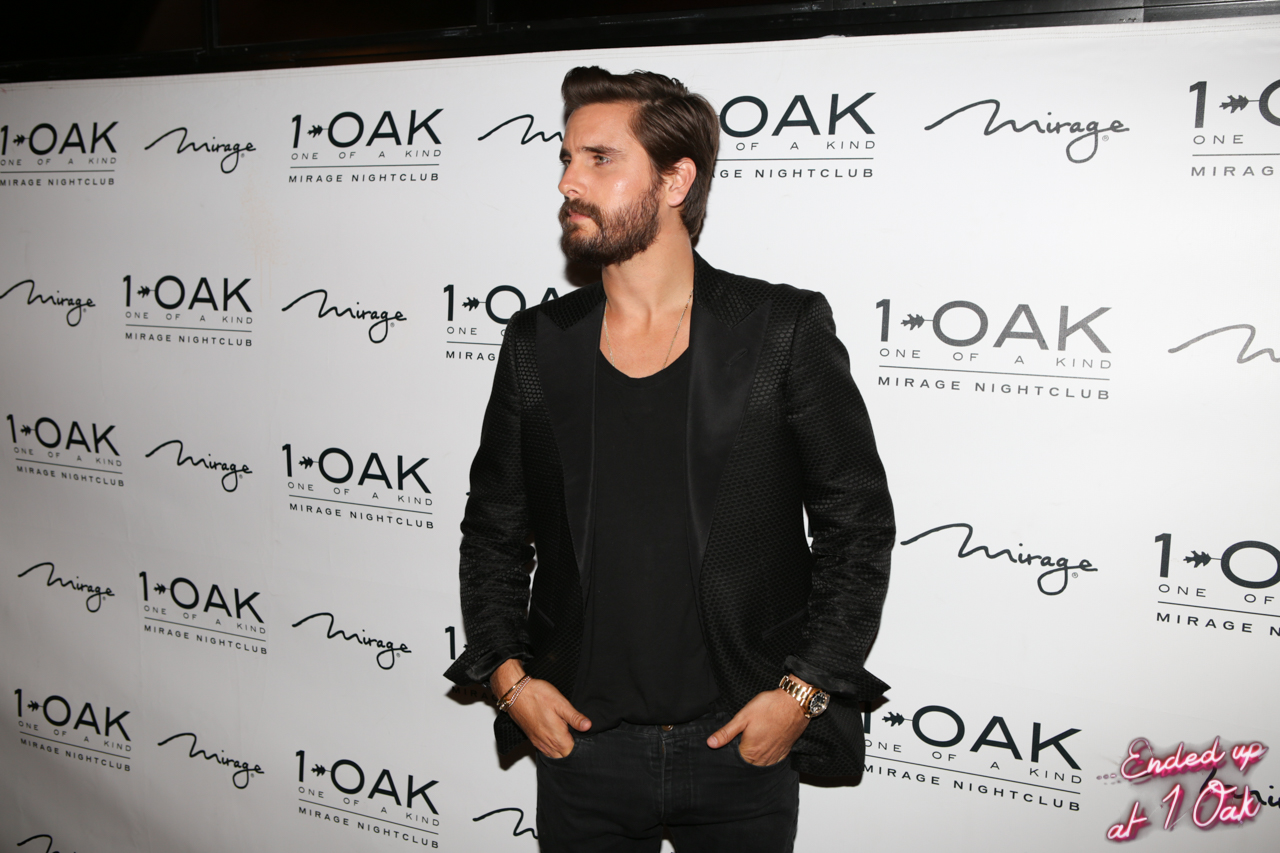The image captures a Caucasian man standing in front of a wall popularly adorned with the repeating text "1-Oak, One of a Kind, Mirage Nightclub." The backdrop, characterized by its black, white, and silver hues with splashes of pink and purple, suggests the setting is a nightclub event, likely indoors at night. The man, positioned centrally in the frame, has dark short hair and a well-trimmed beard and mustache. He is wearing a black V-neck shirt under a black jacket, paired with dark jeans. Accessories include a wristwatch on his left wrist and bracelets on his right. Notably, in the bottom right of the image, the text "Ended Up at One Oak" is visible. His eyes seem light, though indistinct, and he gazes off to the left. The overall scene exudes an elegant, nightlife vibe.